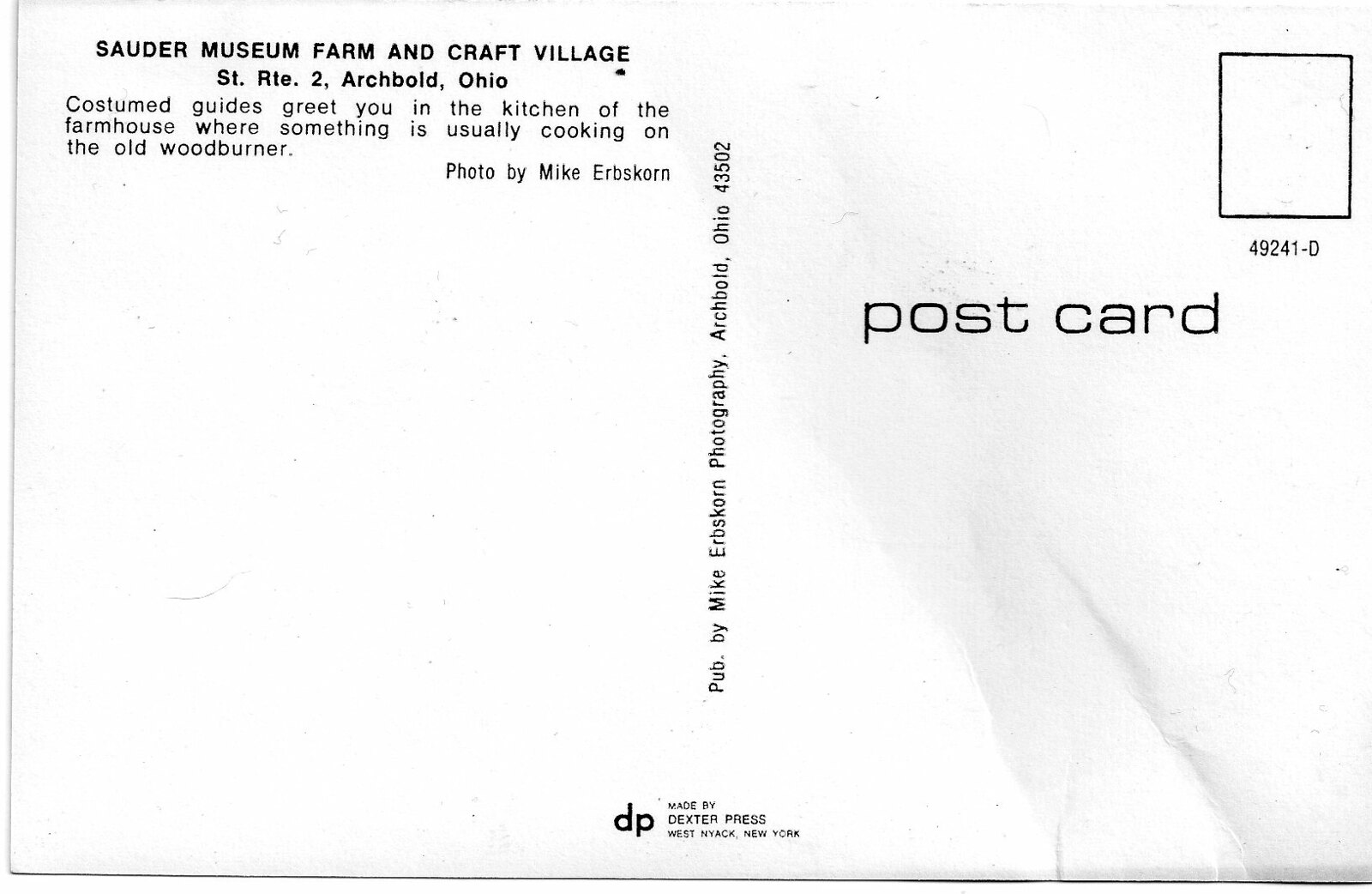The postcard features a white background with a simple black border along the left side and bottom. In the upper right-hand corner, a black outline of a square designates the stamp placement, beneath which are the numbers "49241-D" and the word "POSTCARD" in bold black lettering. The top left corner contains the title "SAUDER MUSEUM FARM AND CRAFT VILLAGE" with the location "ST. RTE 2, ARCHIBALD, OHIO" directly below it. Under this, a paragraph reads: "COSTUMED GUIDES GREET YOU IN THE KITCHEN OF THE FARMHOUSE WHERE SOMETHING IS USUALLY COOKING ON THE OLD WOOD BURNER." Vertically in the middle of the postcard, it states “Published by Mike Erbskorn Photography, Archbald, OH 43502.” Towards the bottom, centrally located text reads "MADE BY DEXTER PRESS, WEST NYACK, NEW YORK." Notably, there is an ink stain starting from the bottom right corner, extending upwards to the left.